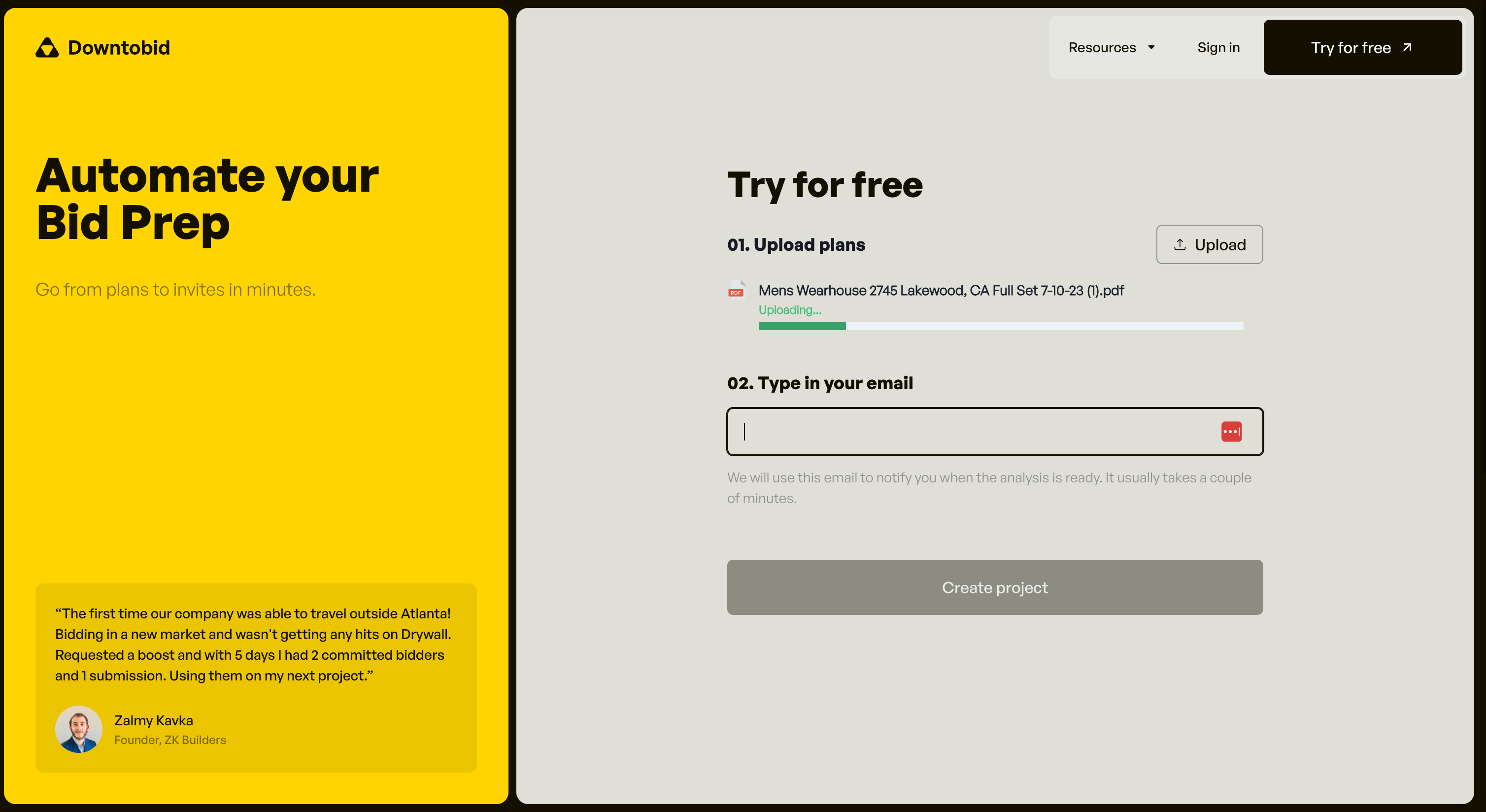In the image, the left section features a vivid yellow background. At the top, bold black text reads "Down Tobin," followed by another bold statement in black, "Automate Your Bid Prep." Below this, in grey letters, is the phrase "Go from plan to invites in minutes."

Beneath this section, there is a testimonial box. This testimonial details how, for the first time, a company was able to travel outside Atlanta to bid in a new market. Initially unsuccessful in securing any hits on drywall, they requested a boost and, within five days, secured two committed bidders and one submission. The testimonial is attributed to Dow Me Corp. 

On the right side of the image, there is a grey box. At the top of this box, the word "Resources" is displayed. Adjacent to this, there is a "Sign In" link. Below it, a black box with the text "Try for Free" is prominently placed. Additionally, the phrase "Try for Free" is repeated in black text just beneath the box.

Under this section, the steps for using the platform are outlined:
1. "Upload Plan" is indicated, accompanied by an upload button. Below the button, it shows a file name and an upload bar with the status "Uploading."
2. The next step says "Type in Your Email," with another text box below. Finally, the left section is concluded with the phrase "Go from plan to invites in minutes" reiterated.